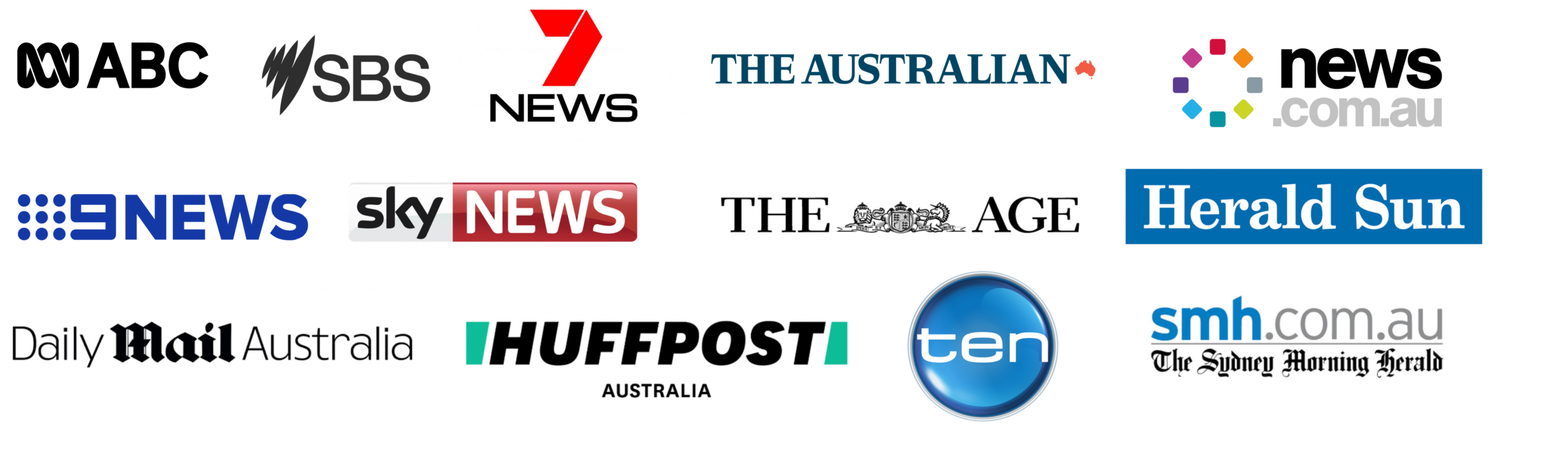This image displays a variety of logos associated with news organizations, including newspapers, news channels, and news affiliates. The first logo features "ABC" set within a horizontally aligned figure-eight shape. Next is "SBS," accompanied by a dynamic scribble-like design to its left. "7 News" prominently showcases a red numeral 7, with the word "News" printed in black. "The Australian" logo is entirely in navy, supplemented by a red emblem beside it.

"Our News" incorporates a multi-colored wheel positioned next to the text, which is located lower on the image. The "9 News" logo is blue and includes dotted elements. The "Sky News" logo presents "News" in red with a white center.

"The Something Age" is presented entirely in black text. "Herald Sun" features a blue rectangular backdrop with white lettering. "The Daily Mail Australia" is noted for its light gray typography, except for the word "Mail," which is prominently rendered in bold, black letters.

"Huff Post Australia" has "Huff Post" in uppercase, dark lettering, while "Australia" is printed smaller. A blue circle contains the numeral "10" in white. Finally, "smh.com.au" is in gray text, with the letters "smh" distinctly highlighted in blue.